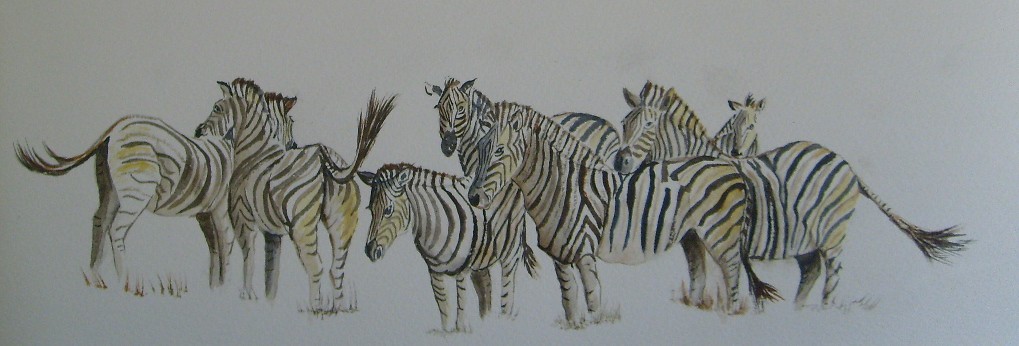This is a detailed illustration of eight zebras against a solid white background. The zebras are depicted in a style that blends realistic and slightly stylized elements, with clean lines suggesting the use of ink or pencil. Seven zebras overlap, creating a dynamic sense of depth, and are mostly positioned facing left or towards the viewer. Two zebras face backward, showing their rump and bushy tails that resemble paintbrushes. The zebras bear black and white stripes with noticeable yellow or brown shading in the darker areas, adding dimension to their bodies. The image features tufts of brown grass near the zebras' feet, although their hooves fade seamlessly into the ground. The arrangement and number of zebras suggest a small group rather than a full herd, capturing a fleeting moment of their natural grace and interaction.